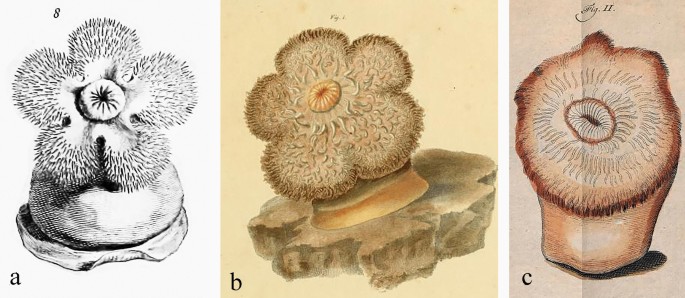The photo depicts three different images labeled A, B, and C. Photo A presents a black-and-white depiction of a five-petaled flower or plant resting on a rounded rock with a thick base. The petals appear prickly, almost like the bristles of a brush, and the center resembles a fleshy or squid-like mouth. In Photo B, the same flower image is shown in color with greater detail; the petals, which seem to have tentacles or hairs, are brown, and the center is orange, evoking the image of lips. The flower is mounted on a larger, beige rock. Photo C portrays a more abstracted rendition of the flower, now appearing more rounded and less detailed. It lacks the distinct petals seen in A and B and has a 2D appearance in shades of red, black, and white. The central feature is still reminiscent of a mouth, surrounded by tentacles or hairs, and rests on a thick base with a large black shadow beneath it.